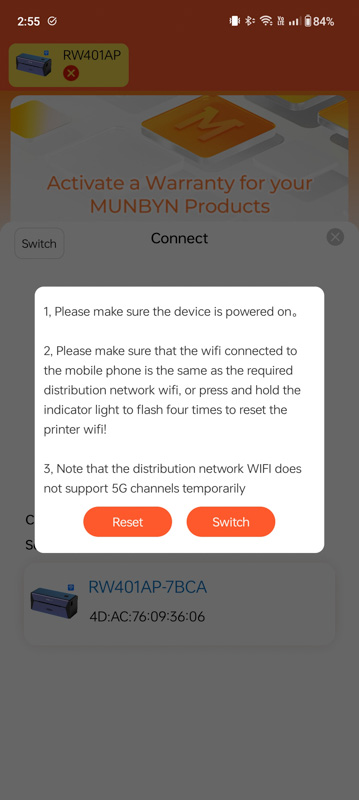The screenshot displays a smartphone interface at 2:55 PM with the battery at 84%, WiFi, LTE, and Bluetooth icons visible at the top-right corner. A white dialog box is centered on the screen containing the following instructions:
1. Ensure the device is powered on.
2. Verify the unit is connected, and the WiFi is linked to the mobile phone.
3. Note that the device does not support 5G.

Below the instructions, there are two buttons: an orange "Reset" button and a "Switch" button. Behind the dialog box, the background shows a website text: "Activate a warranty for your MU-N BYN products" followed by "RW401AP-7BCA" and an image resembling a cubicle or safety puzzle box. Additionally, a switch button, a connect button, and an X button are displayed. Above the "Activate a warranty" prompt, there is another image of the box with the serial number "WRW401AP."